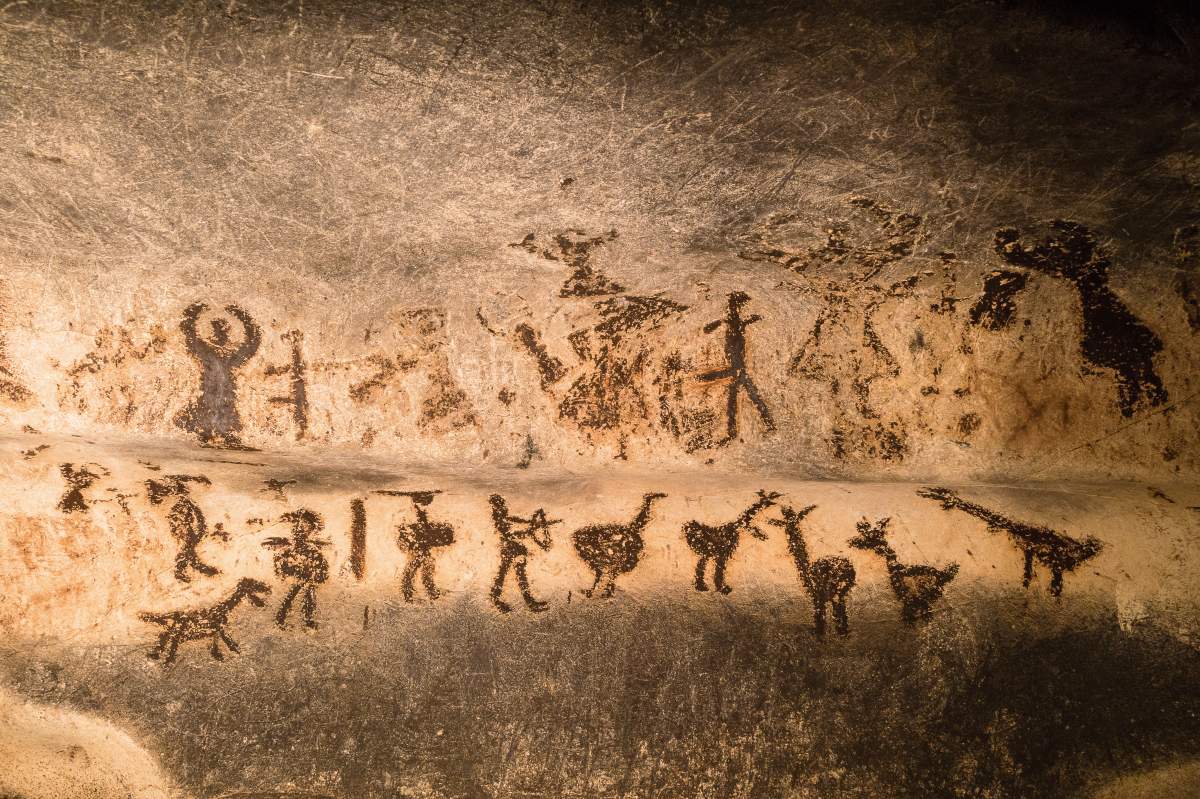The image is a photograph of intricate cave drawings, etched into a rugged stone wall with a rough, textured surface. The photo appears to be taken inside a cave, showcasing a rectangular section about six inches wide and four inches high. The scene is illuminated by some light source, revealing the stunning details of the primitive drawings. The top right and bottom sections of the rock are dark, while the center portion is a lighter cream color, creating a stark contrast.

Across the center of the image, the stone wall features a ledge that both protrudes outward and descends, forming a natural compositional line. Above the ledge and on its surface, rows of dark brown carvings depict a variety of figures. These include stick figure humans, some of whom appear to be dancing with their hands raised or engaged in activities like hunting, evidenced by bows and arrows. Among the humanoid figures are silhouettes of various animals, including what seem to be giraffes, ostriches, dogs, and possibly deer. The interplay of light brown stone and dark brown carvings enhances the visibility of these ancient etchings, offering a striking glimpse into early human artistry and storytelling.